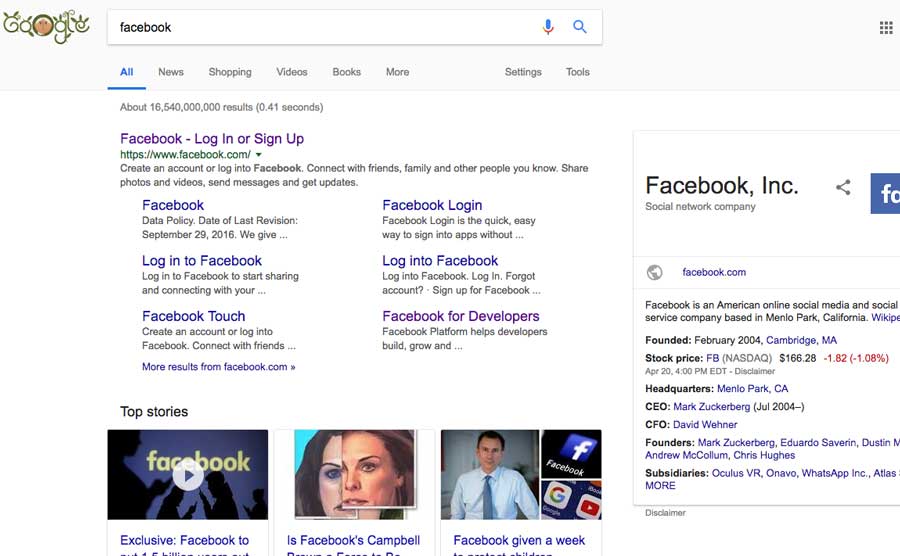The image displays a Google search results page with the Google logo in the top left corner, creatively designed using vine-like elements. The search query entered is "Facebook," and the results are displayed below various filtering options, including "All," "News," "Shopping," "Videos," "Books," "More," "Settings," and "Tools."

The search yields approximately 16.54 million results in 0.41 seconds. The top result, highlighted in purple to indicate a previous visit, is labeled "Facebook - Log In or Sign Up." This is followed by various other login-related links such as "Create an account or log in to Facebook," "Log into Facebook," "Facebook Touch," "Facebook Login," "Login Facebook," and "Facebook for Developers."

On the right-hand side of the page, there is an information panel providing details about Facebook, Inc. It states that Facebook is an American online social media and networking company headquartered in Menlo Park, California, founded in February 2004 in Cambridge, Massachusetts. The stock price is listed as $168.26, down $1.82 or 1.08%. The panel also includes details about the CEO, Mark Zuckerberg, who has held the position since July 2004, and the CFO, David Wehner. The founders are identified as Mark Zuckerberg, Eduardo Saverin, Andrew McCollum, Dustin Moskovitz, and Chris Hughes. The company's subsidiaries, such as Oculus VR, WhatsApp Inc., and Atlas, are also mentioned. A "More" button is available for additional information.

The bottom portion of the image hints at "Top stories" related to Facebook, though these stories are cut off and partially visible at the edge of the page.